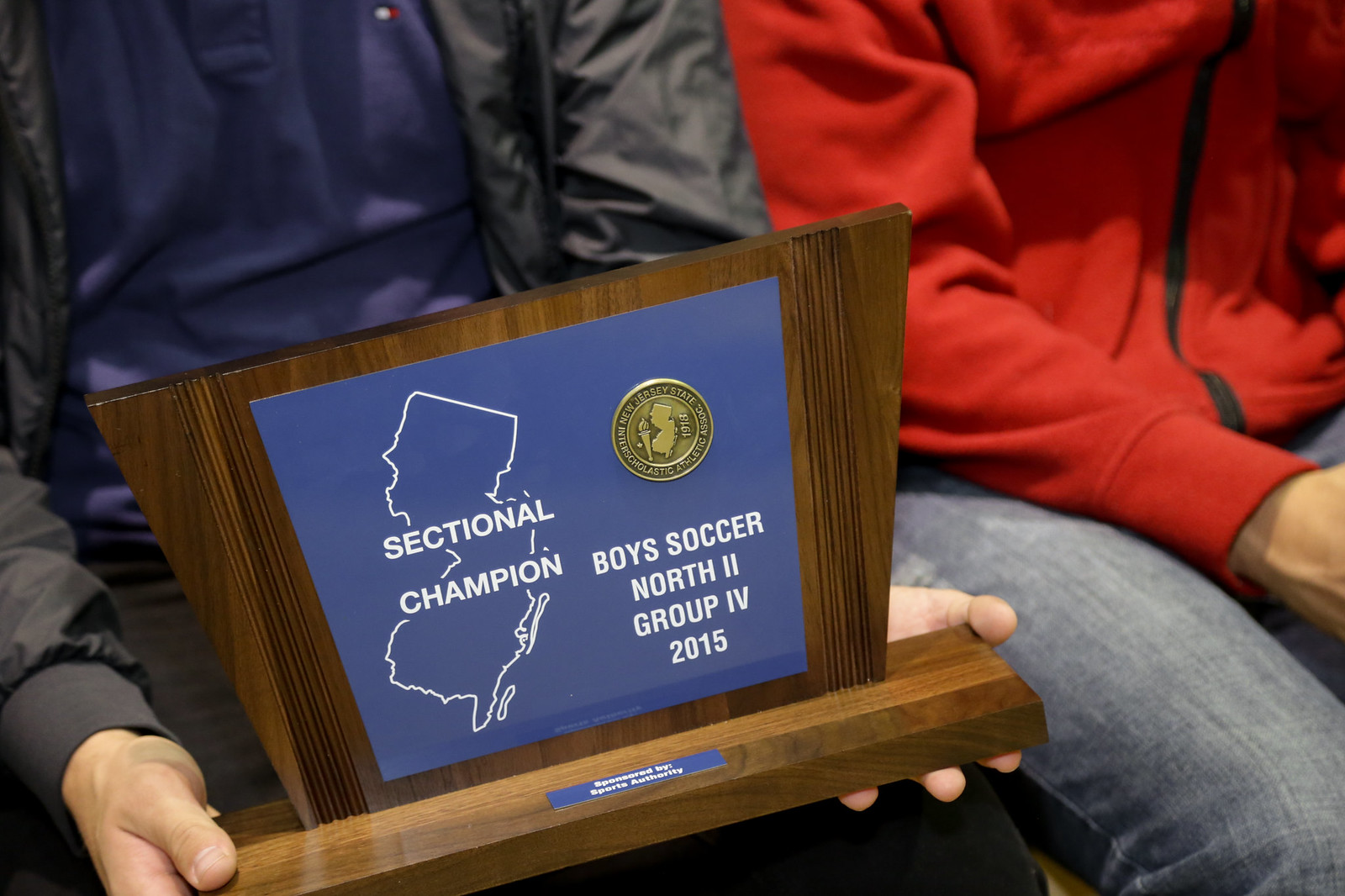The image shows a close-up of an individual holding a uniquely designed trophy, which commemorates a sectional championship. The trophy features a crafted wooden base, adorned with a small, unreadable rectangular blue plaque. Atop the base rests a blue, flat-topped board grooved along its edges. In the center of this board is an outline of New Jersey, emphasizing the geographic specificity of the award. Across this outline, the words "Sectional Champion" are prominently displayed. In the top-right corner of the board, a golden coin-like emblem is attached, inscribed with "1913" and representing the New Jersey State Interscholastic Athletic Association. Below the map, the trophy further specifies the winning event: "Boys Soccer North 2 Group 4 2015". The person holding the trophy is dressed in a jacket with long sleeves and a blue undershirt, while another individual in a red long-sleeved shirt and jeans sits beside them.